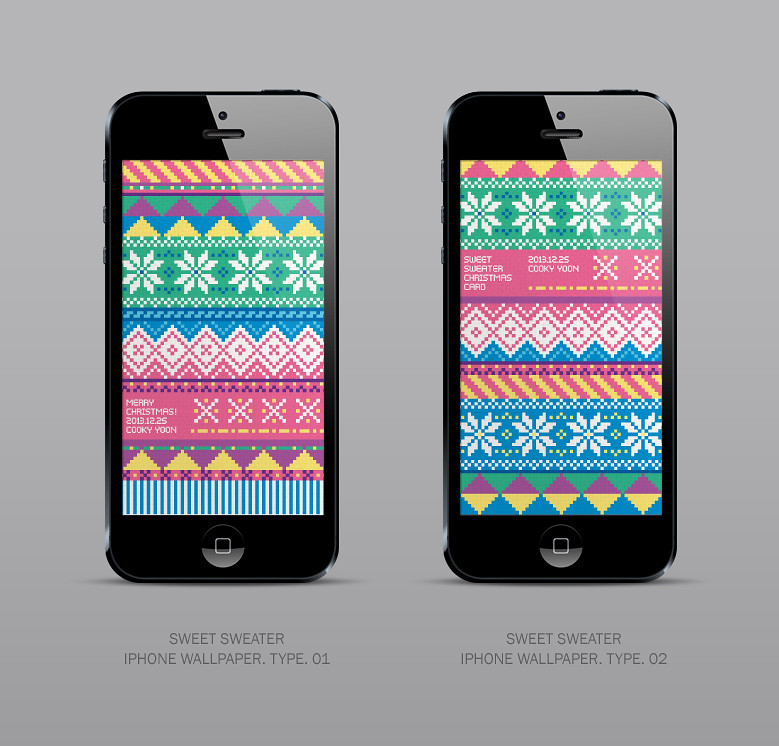This image features two black iPhones, likely older models such as the iPhone 6 or 7, standing upright next to each other. Both screens display a pixelated, Christmas-themed sweater design in various colors such as green, blue, purple, and pink. Despite slight variations in colors and shapes, the patterns on the screens are largely similar. The iPhone on the left has a caption that reads, "Sweet Sweater iPhone Wallpaper Type 01" with text on its screen saying, "Merry Christmas, 2013, 12, 25, Kuki Yoon." The iPhone on the right is captioned, "Sweet Sweater iPhone Wallpaper Type 02" and its screen reads, "Sweet Sweater Christmas Card, 2013, 12, 25, Kuki Yoon." Each phone has a single button at the bottom with a square logo inside and a small speaker at the top, with both screens creatively showcasing the festive 'Sweet Sweater' wallpaper variations.